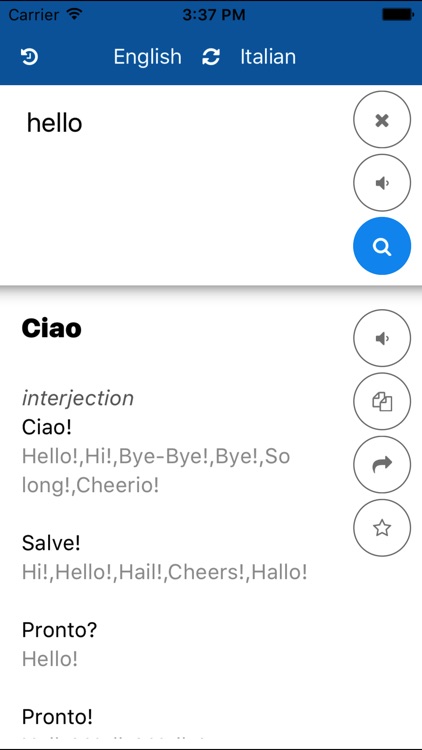This vertical rectangular image appears to be a screenshot from a cell phone, displaying components of a translation or language learning app interface.

At the very top, in a small horizontal black area, the following elements are organized from left to right: the word "carrier" in black font, the time displayed as "3:37 PM" in black font, and a battery icon, also in black, indicating a full charge.

Below this is a blue horizontal bar featuring white text which reads "English" on the left, accompanied by two circular arrows forming a loop, indicating a translation function, and "Italian" on the right.

The next section, taking up about a third of the image, is a white horizontal area. Here, the word "hello" is displayed in black, lowercase letters. To the right of this text are three circular icons: the top one with a gray X, the middle one with a speaker icon (indicating an option to play audio), and the bottom one with a blue background and a white magnifying glass (suggesting a search function).

The largest vertical section of the image begins with the bold black word "ciao" (the Italian translation for "hello"). Underneath "ciao" is the word "interjection" in regular black font, followed by a slightly bolded "ciao!" along with its various English equivalents: "hello!", "hi!", "bye-bye!", "bye!", "so long!", and "cheerio!".

Further down, another slightly bolded term, "salve!", is listed with corresponding translations: "hi!", "hello!", "hail!", "cheers!", and "hello!" spelled as "hallo!".

Following this, the word "pronto?" (indicating a question for "hello?" used in answering phone calls) is slightly bolded, with its translation "hello!" listed beneath. Another slightly bolded "pronto!" (used as an exclamation for "hello!") is also included.

A very thin black horizontal line appears at the bottom of this section. 

On the far right-hand side of the image, organized in a vertical column, are four icons inside circles, all in gray font: a speaker icon, a two-paper icon (probably for copy functionality), a right arrow (indicating forward or next), and an unfilled star (likely for saving or favoriting).